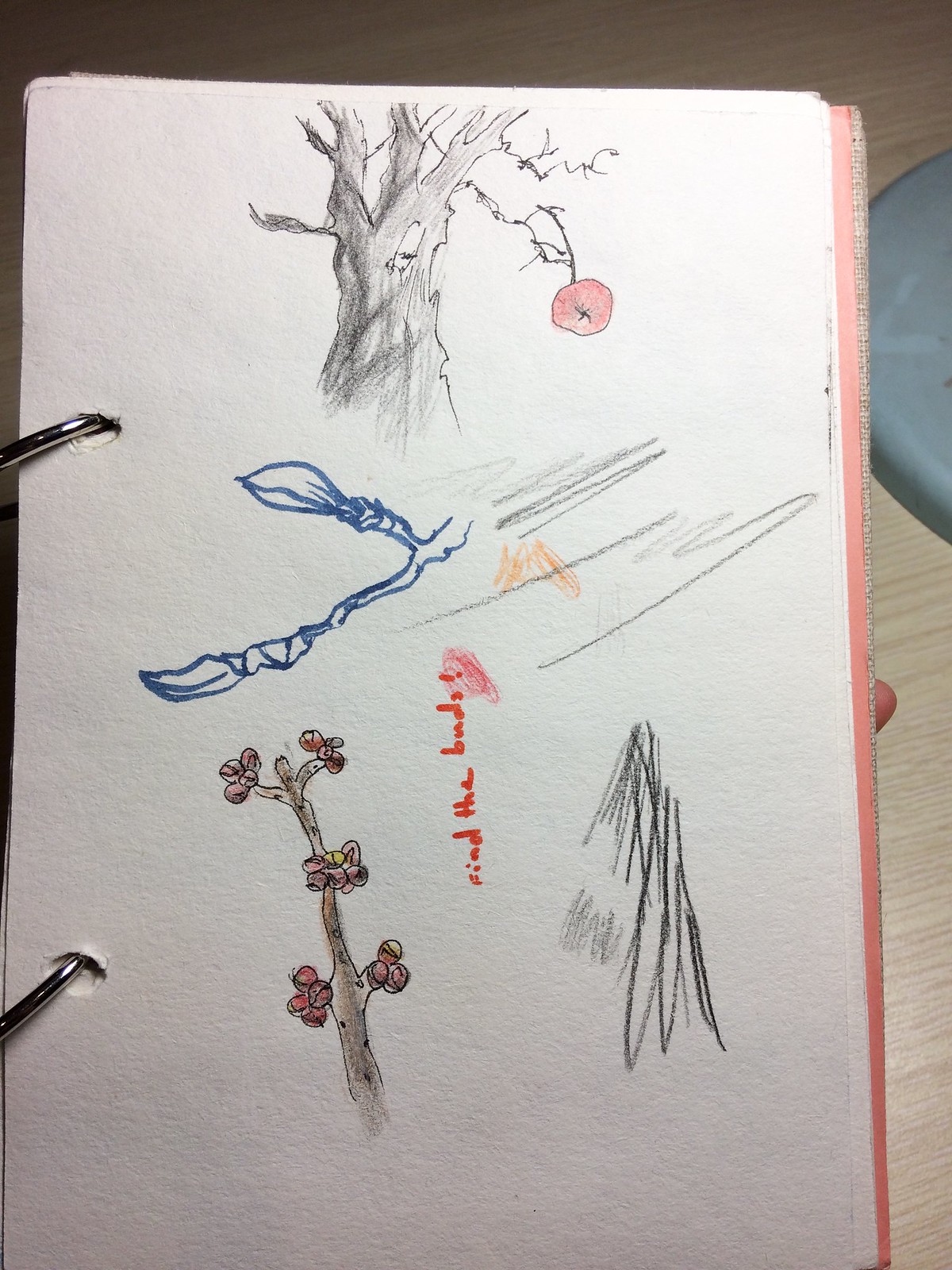A photograph captures a textured sketch pad, possibly being held by someone, as a finger is slightly visible behind it. The image prominently features the sketch pad, which is roughly 8.5 by 11 inches and held together with two metal rings from a binder. The drawing on the pad is intricate and partially colored. At the top, there is a pencil sketch of a near-barren tree, evocative of the Wizard of Oz’s trees, with spindly branches and, hanging from one of them, a single prominent red apple or berry. Below this tree, rendered in blue marker, is a branch with budding blossoms. Further down is another branch drawn in brown, adorned with red flower buds. Throughout the pad are various scribbles in pen and pencil. In the middle, written in red ink, are the words "Find the Buds!" The photo's background hints at a wooden floor, a possible cushion, and parts of a grey object and table.